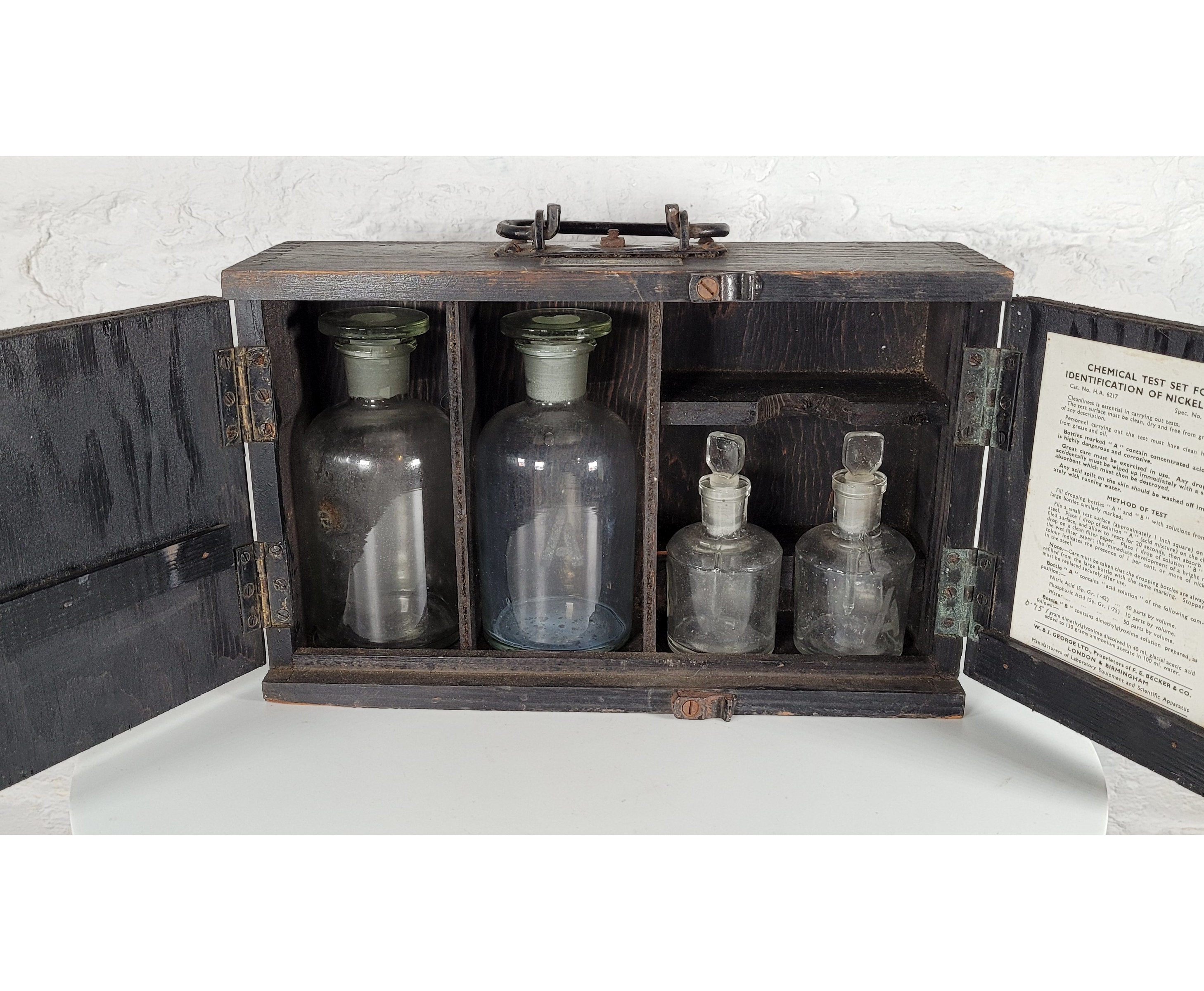The image depicts an antique wooden cabinet with a handle on top, designed to be portable. The cabinet is horizontally aligned and rectangular in shape, featuring two hinged doors that are open to reveal its contents. The wood is dark and worn, with darker grains running through it, giving it a distinctly aged appearance. Inside, the cabinet's shelves are a brown color, while the interior of the doors appears black.

Inside the cabinet, there are four old, dirty, and dusty glass containers that seem to date back to the 1800s. On the left side, there are two taller bottles, approximately 8 to 10 inches high, each with glass stopper lids and separated by a wooden divider. On the right side, there are two shorter glass bottles, also with glass caps, and another wooden separator. The right door of the cabinet bears a white paper sign with black text that reads "Chemical Test Set Identification of Nickel," accompanied by a lot of fine print below the heading.

The entire setup is placed on a white round table, and the background features a textured white wall, providing a stark contrast to the dark, antique wood of the cabinet.